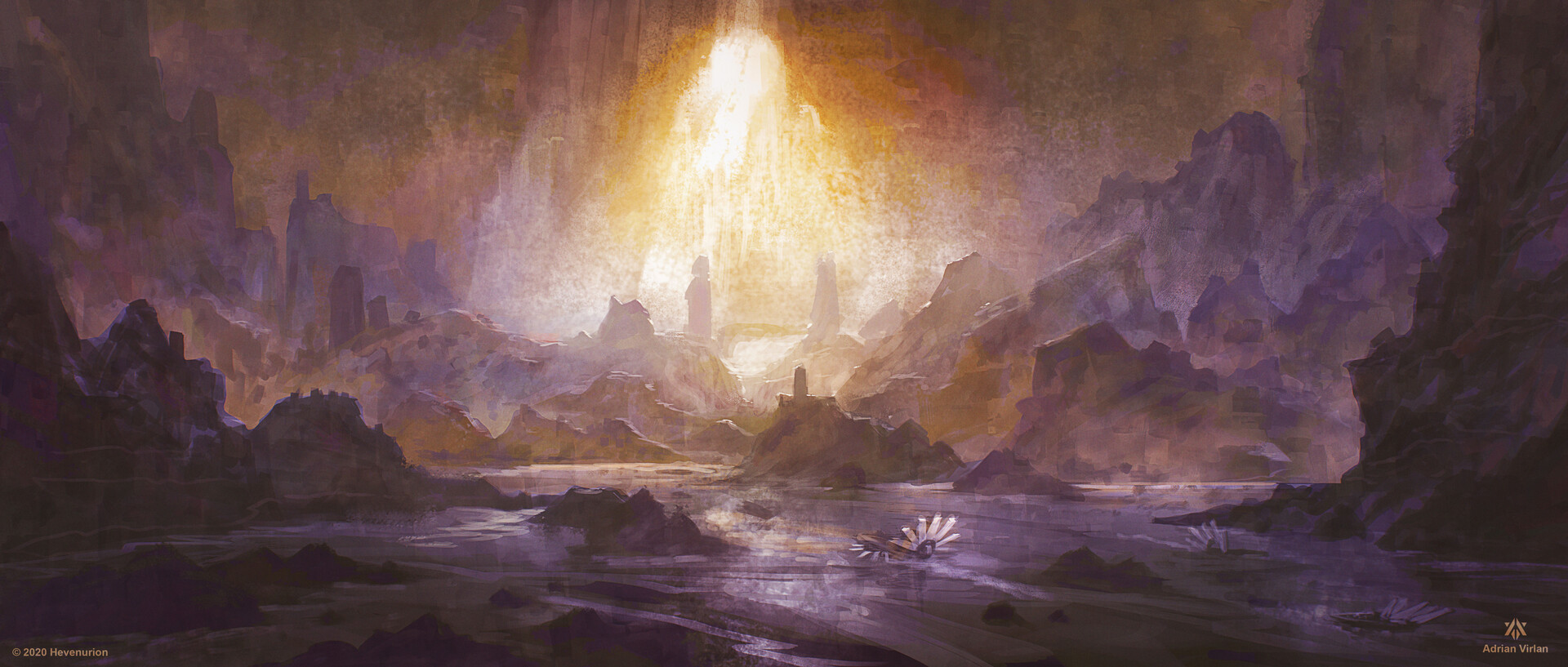This rectangular painting by Adrienne Verlan, measuring approximately six inches wide and two inches high, presents a dramatic and atmospheric cave landscape. Dominated by hues of yellows, blacks, whites, grays, purples, and mauves, the dark edges contrast starkly with the bright beam of yellow-orange light streaming down from an opening in the top center. This light illuminates the rocky interior, with built-up rocks and stalagmites flanking the scene. The landscape appears hazy and grayed out, adding to the mysterious ambiance. Notable details include what seems to be a dead bug or flower in the bottom middle, enhancing the depiction of the cave's floor. The artist's signature and copyright information, marked as Hevennerion 2020, are located in the lower corners, with the name Adrienne Verlan and a stylized "AV" monogram in light brown print on the bottom right. The painting evokes a sense of intrigue, portraying a misty and ethereal subterranean world.